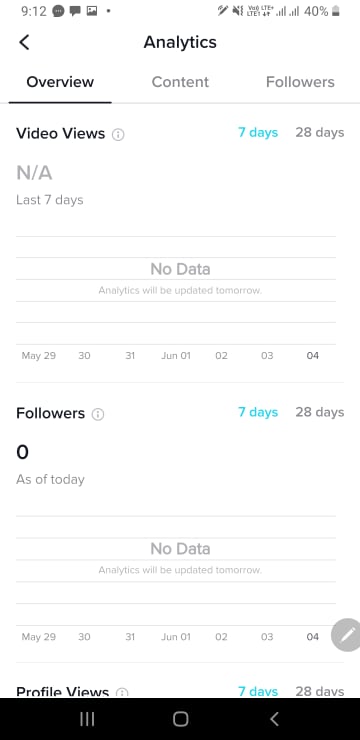Screenshot of a mobile phone displaying the "Analytics" page within the settings app. The page is on the "Overview" tab, with additional tabs for "Content" and "Followers" visible but not selected. The screenshot is taken at 9:12 a.m. The phone's battery is at 40%, and there are several notification icons visible at the top of the screen. 

The "Analytics" page features sections for "Video views," "Profile views," and corresponding analytics data. Notable text includes:

- "Analytics"
- "Overview," "Content," "Followers" tabs
- "Video views" in blue font
- "7 days" in blue font, "28 days" in gray font, "N/A" below that
- "No data," indicating that analytics will be updated tomorrow
- A series of dates beginning with May 29th

The background is white, with black and gray text, and occasional blue font for emphasis. There are currently no data displayed for "Video views" and "Profile views."